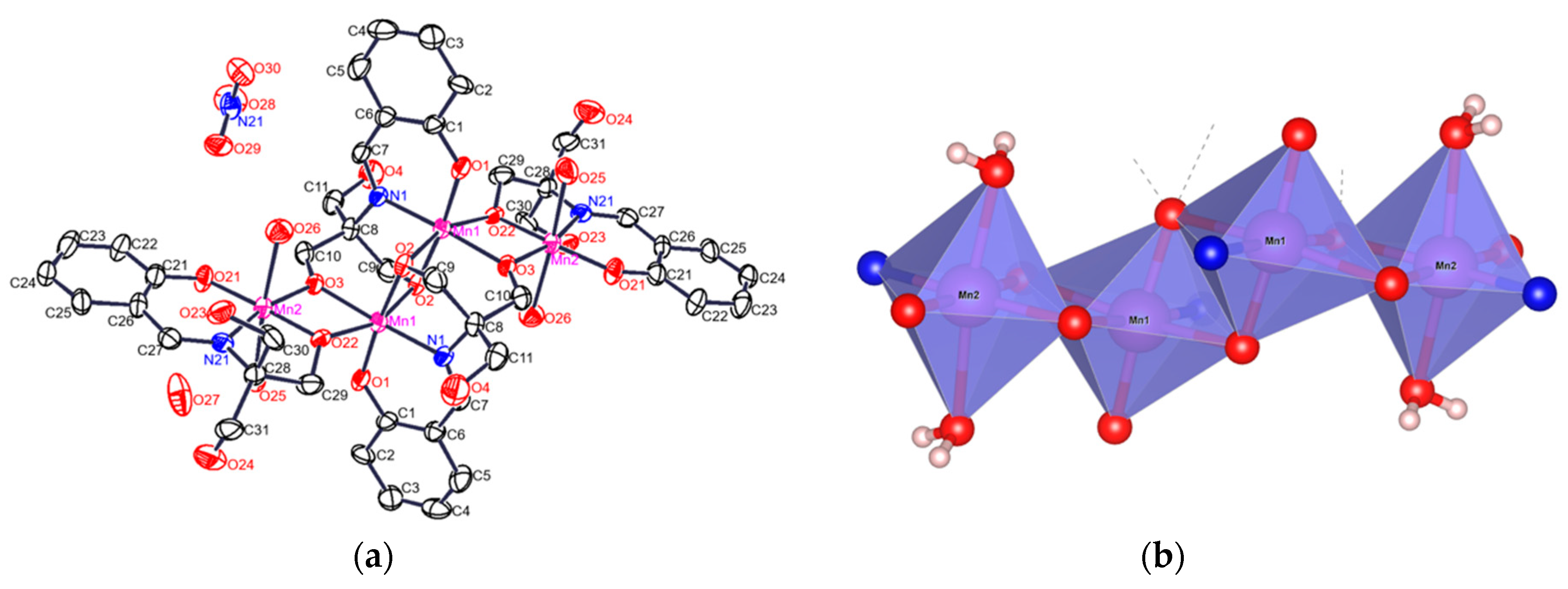The image is divided into two parts, labeled A on the left and B on the right. Part A features a complex diagram consisting of black lines that form diamond and square shapes, resembling a spiderweb. The diagram includes several colored annotations: black font lowercase serif letters, red circles, blue circles, and pink circles, each with a unique identifier. The annotations range from C1 to C30 and O1 to O30, with C identifiers in black, O identifiers in blue, and numbered dots in red and blue. Part B displays four three-dimensional purple diamond-shaped prisms, each with red and blue balls located at certain points. These prisms have red and blue dots, as well as some pink dots. The prisms are labeled MN1 and MN2, with MN1 repeated twice in the middle. The entire right side offers a distinct geometric contrast to the detailed, annotated network on the left.